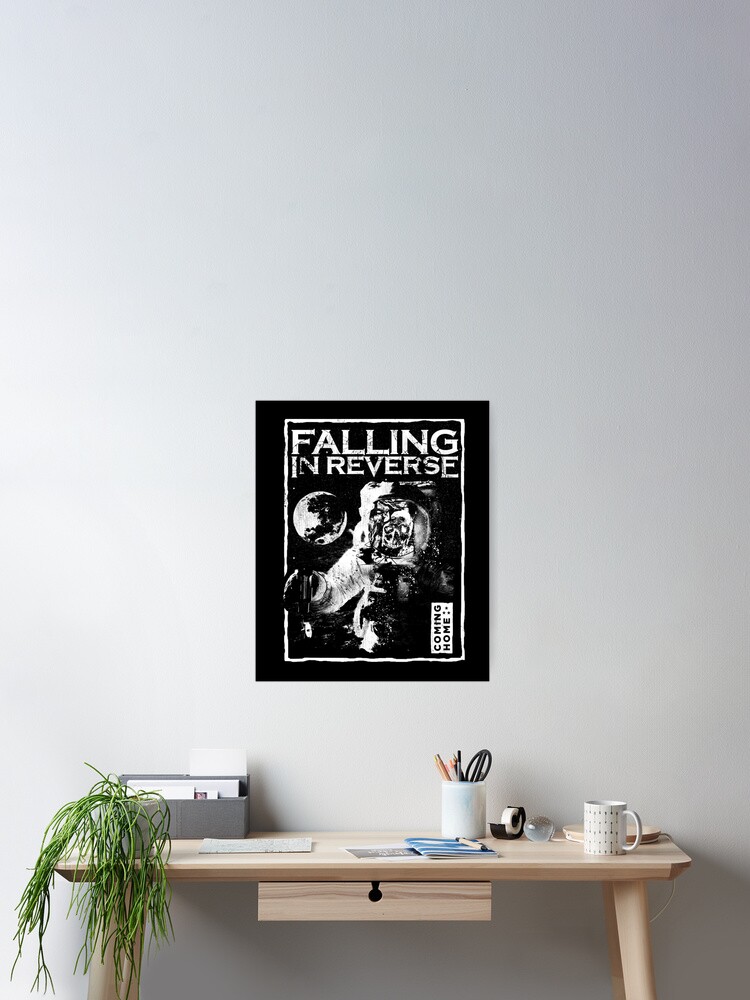The photograph, taken indoors, depicts a simplistic, well-organized workspace that one might see in an interior design magazine. At the center right-bottom of the image is a small wooden desk, likely made of white pine, against a gray wall. This desk features a single drawer beneath its surface. Atop the desk, a variety of items are neatly arranged: a white cup containing pens, pencils, and scissors is present, along with a small tape dispenser positioned to its right. A marble or glass object is situated further right, followed by a white coffee mug. A long, thin white desk lamp is placed behind the coffee mug. On the left side of the desk, there is a gray mail holder with a potted plant in front of it, its green leaves drooping elegantly over the desk's edge. 

Above the desk hangs a prominent black and white poster. This poster, with the words "Falling in Reverse" at the top and "Coming Home" at the bottom, portrays an astronaut in black and white, his skull visible through his helmet, possibly floating in space with celestial bodies in the background. The cohesive and thoughtfully curated elements of the desk and surrounding area contribute to a minimalist yet inviting aesthetic.